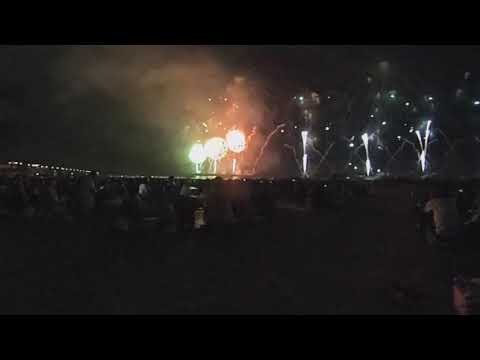The image captures a nighttime outdoor fireworks display. The bottom half is predominantly black, filled with the silhouettes of people standing and watching the spectacle. The center and upper parts of the image feature bursts of colorful fireworks, with greenish, reddish, and yellowish hues forming spherical shapes. There is noticeable smoke in the upper left quadrant, spreading from the pyrotechnic display. On the right side of the image, three light trails, possibly from additional pyrotechnics, create a series of bright white sparks rising into the night sky. Overall, the photograph is dark and somewhat blurry, with most illumination derived from the fireworks and light trails. Street lights appear as a straight line of lights from left to right, adding subtle background illumination. The dynamic colors and movement of the fireworks contrast starkly against the deep black backdrop of the night.